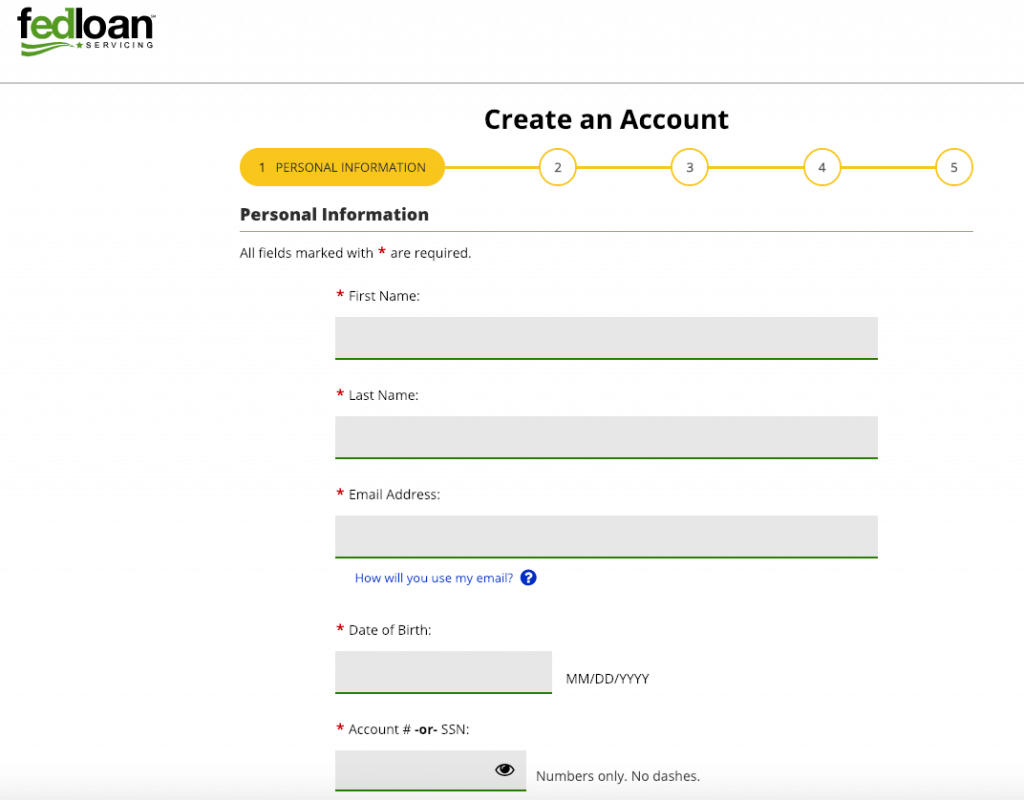This screen capture from a website features a clean, white background with multi-colored text. At the top, "Fed Loan Servicing" is prominently displayed, using a mix of green and black font. Below the "Fed" portion, there are two green wave-like lines. Moving downward, a thin gray line separates the header from the content below. Underneath this line sits a gold bar containing black text, labeled "1. Personal Information."

Following this gold bar, there are white circles with black numbers, encircled in gold, sequentially numbered from "2" to "5." Beneath this, the words "Personal Information" are displayed in black font. A statement follows in black text, clarifying that "all fields marked with a red asterisk * are required."

There are several text fields designed for user input, each presented as gray boxes with a thin green underline and a red asterisk preceding them to indicate mandatory fields. The first field is labeled "First Name," followed by "Last Name," and "Email Address." Directly below the email address field, a blue text link reads "How we use my email," accompanied by a blue circle containing a white question mark, providing additional information.

Further down, there is a "Date of Birth" field formatted in black text as "MM/DD/YYYY." Finally, the "Account Number or SSN" field is labeled with a small black eye icon to indicate visibility or security settings and is followed by gray text advising, "Numbers only, no dashes."